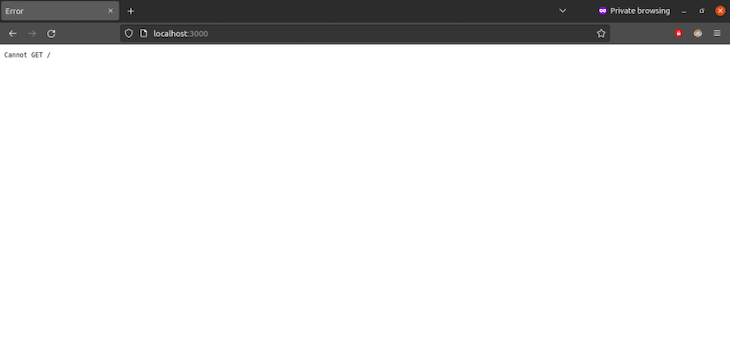The image showcases a web browser's top interface within a private browsing session. The background of the browser is predominantly black. 

- **Top Left Corner:** 
  - There's a single tab labeled "Error" in white text against a grey background.

- **URL Bar:**
  - Centrally positioned at the top, featuring a URL that reads "localhost:3000" in white text.
  - To the left of the URL, there are browser navigation icons such as Back, Refresh, and possibly a Preview button.

- **Error Message:**
  - Directly below the URL bar, there is an error text in black font on a white background, stating, "Cannot GET /".

- **Private Browsing Indicator:**
  - Towards the top right, a blue circle containing a white mask icon indicates private browsing mode.
  - Next to this icon, the words "Private Browsing" are displayed in white text.

- **Browser Controls:**
  - On the top right, there are the typical browser control buttons: 
    - Close (red)
    - Maximize
    - Minimize
  - Below these controls, there's a red shield icon with a white lock, likely indicating a security feature or an SSL issue.

- **Dropdown Menu:**
  - The top right also includes a dropdown menu, though its contents are not specified in the caption.

The overall image seems to depict a webpage that could not be loaded, showing an error message within a private browsing window, with various interface elements described.